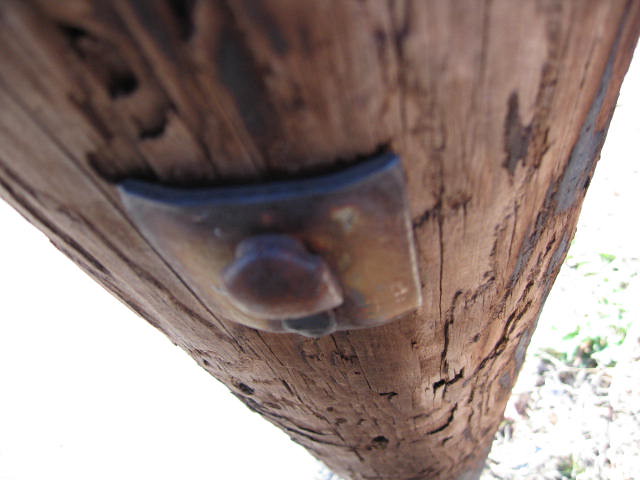This close-up photograph captures a weathered brown wooden telephone pole from a downward angle, emphasizing its central position in the frame. The pole itself is a large, weathered brown wood structure with a metal bolt and a rusted rectangular metal piece attached to it. This rectangular metal piece curves to fit the curvature of the pole. In the center of the metal piece, a round metal object protrudes. The scene is brightly lit, likely taken outdoors in the middle of the day, washing out much of the background detail. On the left-hand side of the pole, the ground is almost completely white, while on the right-hand side, some oversaturated vegetation and dirt are faintly visible. The image is devoid of any text, people, or signatures, focusing entirely on the interplay of light and the textures of the wooden pole and metal elements. The colors in the image range from shades of brown, black, gray, to white and hints of green.